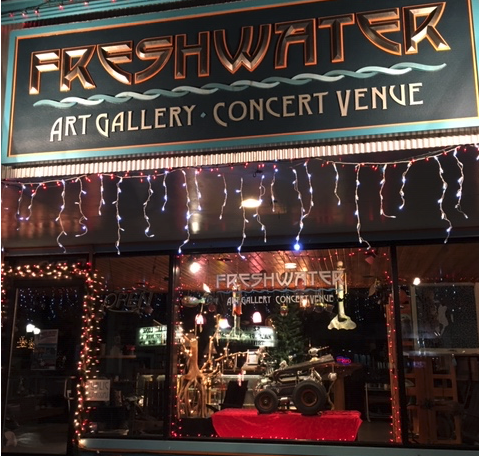The photograph depicts the exterior of the "Freshwater Art Gallery and Concert Venue." Centrally placed at the top of the building's all-glass facade, there is a prominent horizontal rectangular sign with a black background, adorned with gold lettering and blue and gold trim. This sign reads "Freshwater," with a subtitle in a similar decorative style stating "Art Gallery. Concert Venue." Below this sign, festive Christmas lights hang down in vertical strings, creating a sparkling, icicle-like effect around the entrance, indicating the season is around Christmas time.

The glass wall, framed in black metal, bears the same name "Freshwater Art Gallery Concert Venue" in white lettering at its center window. Through the slightly reflective glass, one can discern a red table prominently positioned with a small, four-wheeled remote control car atop it. Various stools and pieces of abstract art are faintly visible inside, though the reflection from the Christmas lights makes the interior contents somewhat difficult to distinguish. An unlit "open" sign further accentuates the welcoming but quiet ambiance of this artistic space.